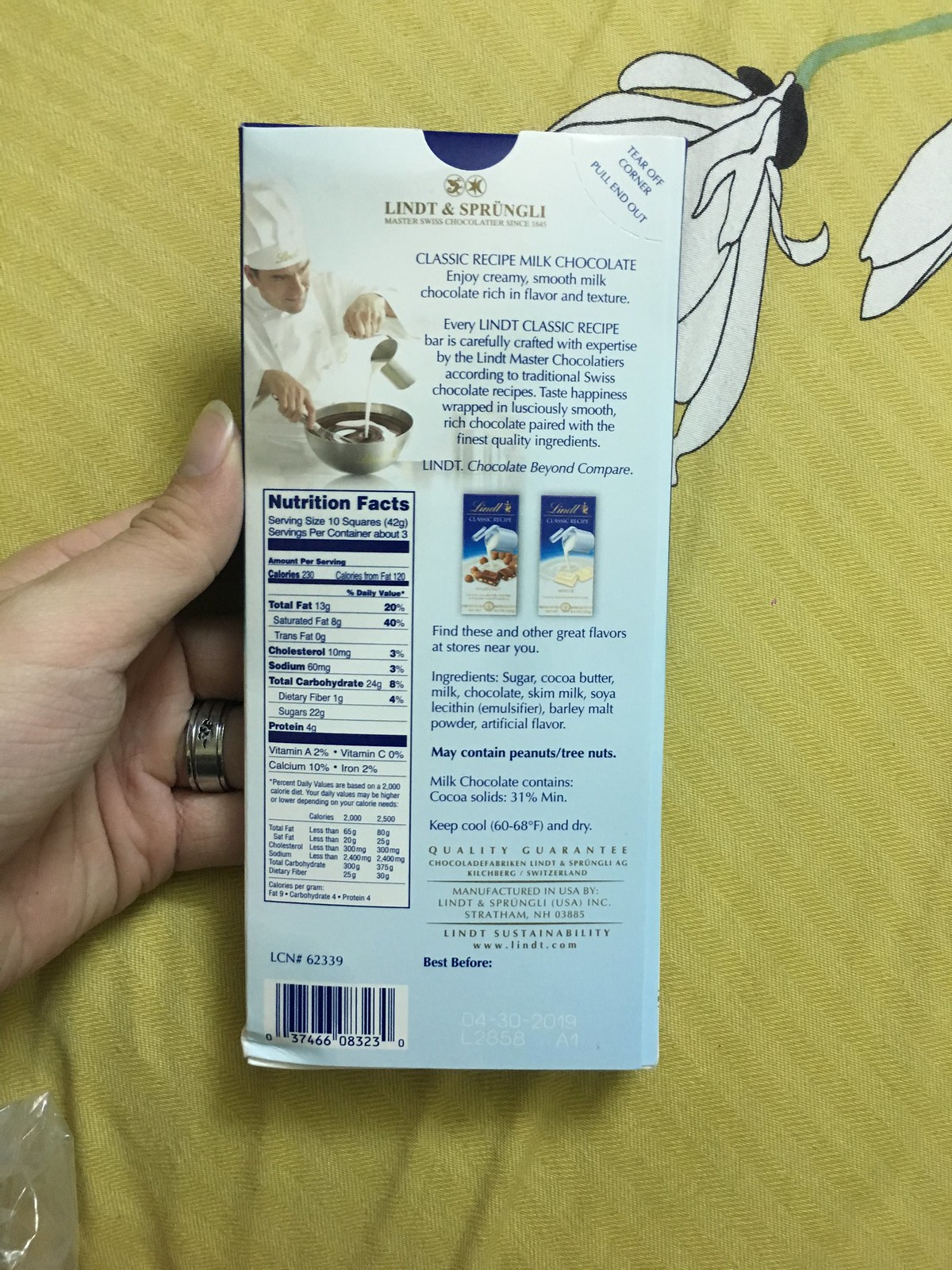In the image, we see a hand with a silver wedding ring holding a light blue box of Lindt classic recipe milk chocolate against a yellow background. The box prominently features a meticulously drawn white flower with a green stem on the right. At the top of the box, "Lindt" is written, and below it, there are detailed nutritional facts on a white background with blue square lettering indicating information about total fat, saturated fat, and trans fat.

On the left side of the box, an illustration depicts a master chocolatier in a white chef's uniform and hat, pouring milk from a white container into a silver bowl filled with dark chocolate, mixing it with a spoon. The text nearby highlights the classic recipe's promise of creamy, smooth milk chocolate rich in flavor and texture. The box's back describes the ingredients, including sugar, cocoa butter, milk chocolate, skim milk, soya lecithin (an emulsifier), barley malt powder, and artificial flavor, with a note that it may contain peanuts and tree nuts, and specifies that the chocolate contains a minimum of 31% cocoa solids. The text also invites consumers to "taste happiness" crafted by Lindt's master chocolatiers according to traditional Swiss recipes. A barcode can be seen in the bottom left corner of the box, along with instructions to keep the chocolate cool and dry.